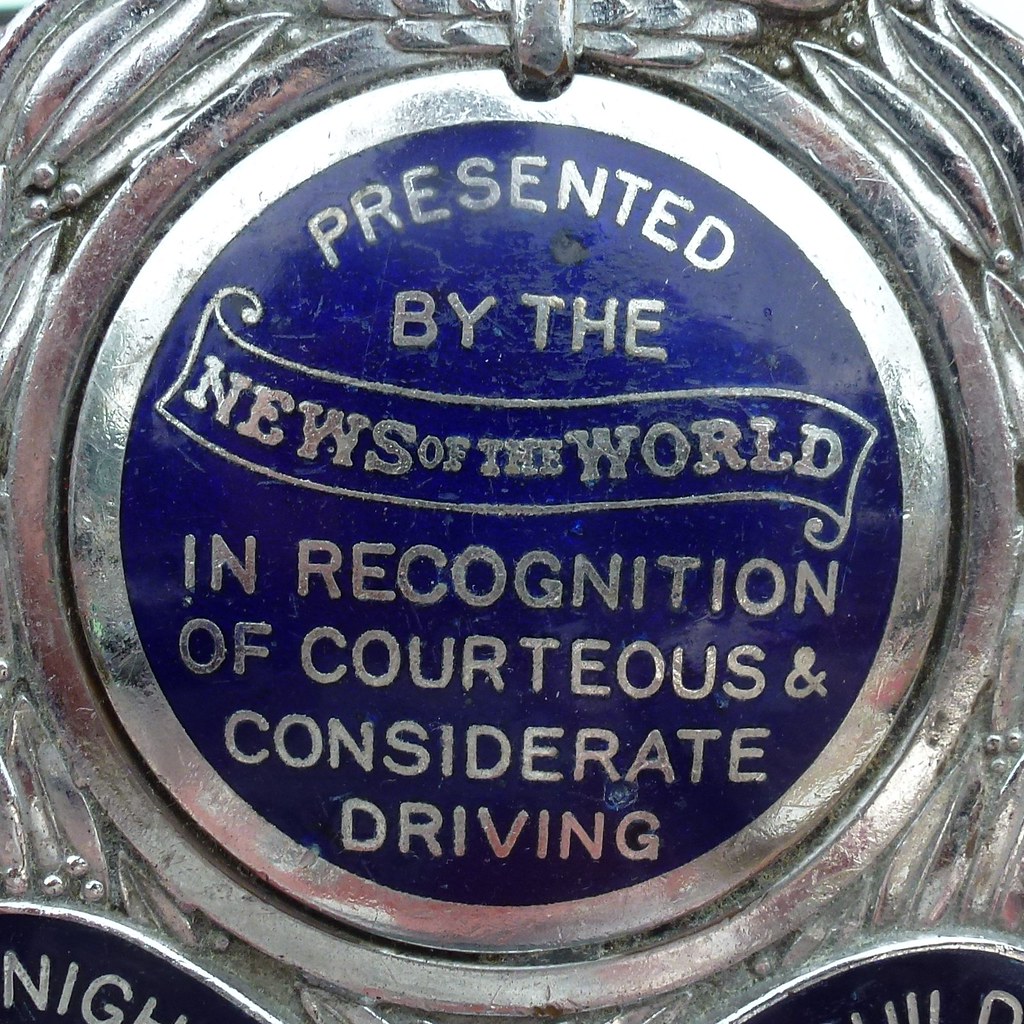The image depicts a very close-up view of a circular metallic medal or award with intricate designs and patterns. The medal appears to be crafted from silver or aluminum, with a textured outer portion featuring a motif that resembles carved or molded leaves. The central area of the medal includes a concentric circle design with an outer ring surrounding a royal blue background. 

In the center, the text "Presented by the" is inscribed at the top, followed by "News of the World" on a stylized floating banner in the middle. Below the banner, the inscription continues with "In recognition of courteous and considerate driving," all in capital letters. The outer portion of the medal is detailed with two additional semicircular sections at the bottom corners, each displaying partial letters within a black background— "N I G H" on the left and "W D" on the right. The medal is worn and bears several scratches, hinting at its age or frequent handling. 

Overall, the medal is presented in a square close-up image, emphasizing its detailed craftsmanship and the significance of its inscriptions.